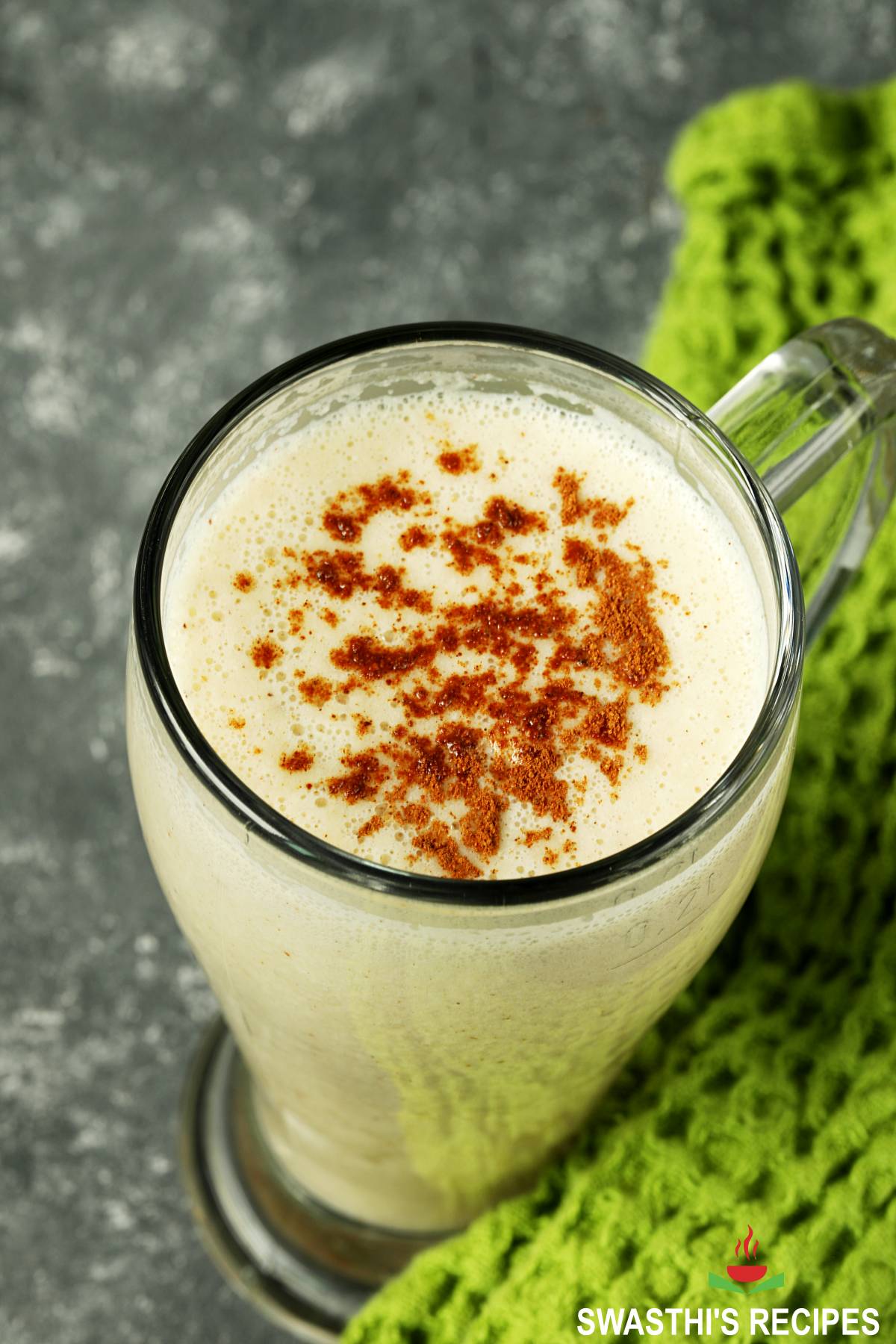The photograph captures a clear glass mug with a handle, filled to the brim with a creamy, frothy beverage that appears to be a latte or possibly eggnog. The drink is topped with a generous sprinkle of cinnamon, adding a warm touch of spice. The mug is centered on a countertop of flecked black and white stone, with a bright green knitted fabric—likely a tablecloth—visible on the right-hand side, lending a cozy atmosphere to the scene. In the bottom right corner, the image features the text "Swasti's Recipes" in white font, accompanied by a red steaming cup and green leaves logo. The mug is sharply in focus, while the background elements remain slightly blurred, emphasizing the inviting texture and presentation of the drink.